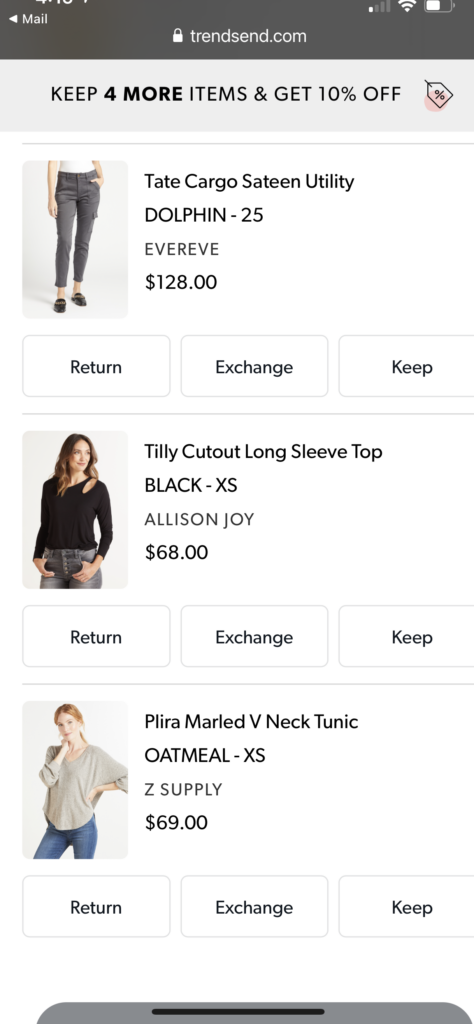The image depicts a digital screen, possibly a shopping app or website, displaying a detailed order summary from trendsend.com. 

At the very top, the interface features a back arrow icon next to the name "Mel," along with status icons for Wi-Fi connectivity and battery percentage. A small lock symbol signifies a secure connection.

Below the header, a promotional message offers a 10% discount for keeping four or more items. The page then lists various clothing items available for purchase, each accompanied by a clear image, description, size, brand, and price.

The first item shown is the "Tate Cargo Satin Utility Dolphin 25" pants, priced at $128, with an image displaying the pants. Buttons for return, exchange, or keep are available.

Following this, the "Tilly Cutout Long Sleeve Top" in black, size extra small from the brand Alice and Joy, is listed at $68. The image alongside shows a woman wearing the black long sleeve top, with options to return, exchange, or keep.

The last item displayed is the "Plyra Marled V-Neck Tunic" in oatmeal color, size extra small from Z Supply, priced at $69. An image of a woman wearing the light oatmeal-colored sweater is featured, along with buttons for return, exchange, or keep.

The entire page has a clean design with a white background and black text, making the information easily readable.